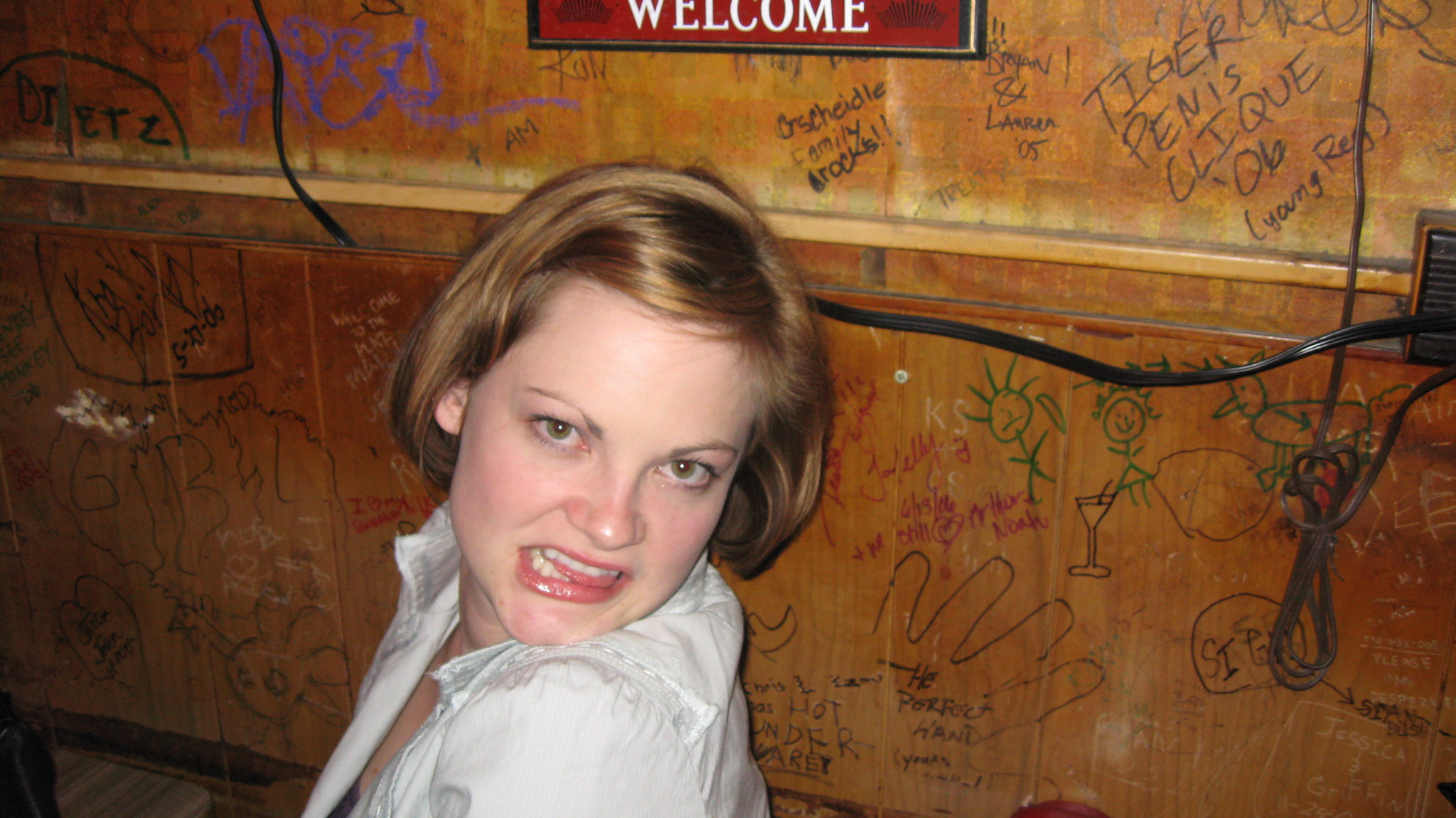The image captures a young woman, likely in her early 20s, with strawberry blonde hair and thin eyebrows. She is seen from the shoulders up, making a playful expression with her mouth open and her tongue sticking out between her teeth. She is wearing a white shirt or jacket and facing the camera head-on. The background features an old wooden panel wall extensively vandalized with various drawings and graffiti in multiple colors, including black, red, green, and purple. Notable illustrations include handprints, martini glasses, and stick figures. A prominent red and white sign that reads "Welcome" is partially visible at the top. Alongside the wall, an electrical outlet with a cord hanging down is also noticeable. The overall setting appears to be a bar or a casual establishment with a heavily doodled wall.